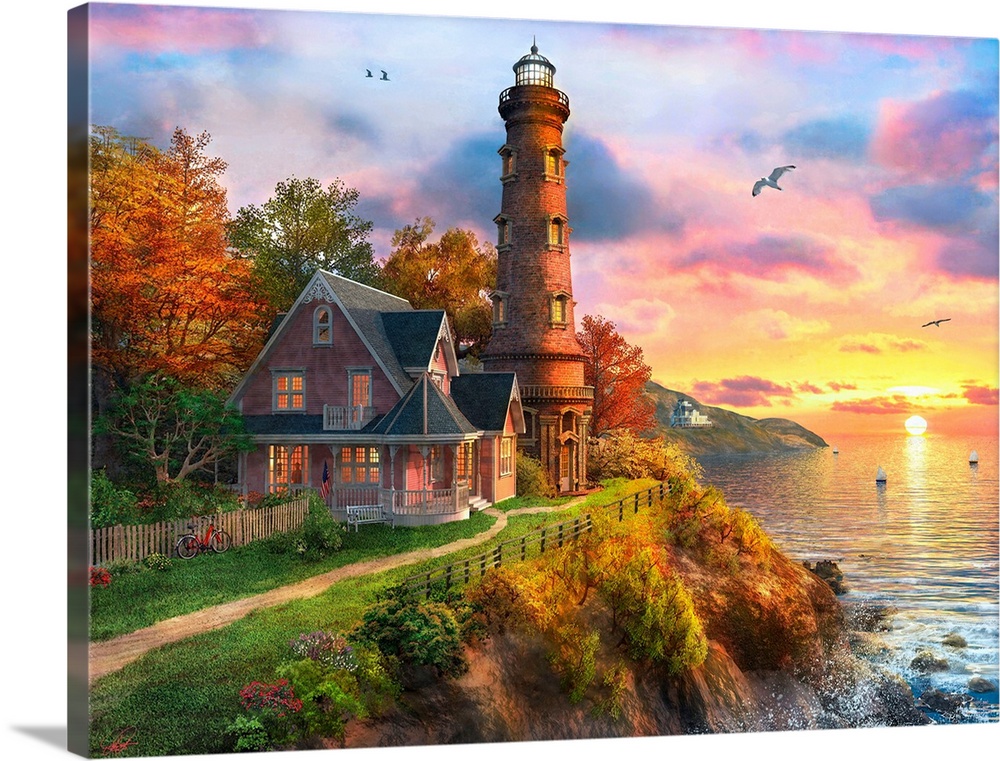The image is a detailed canvas painting showing a serene coastal scene at either sunrise or sunset. The canvas, slightly tilted towards the camera, reveals a beautiful two-story red brick house with an attic, set against a breathtaking backdrop of blue, purple, and yellow hues in the sky. To the right of the house stands a tall red brick lighthouse with multiple yellow windows and a glass-enclosed top, suggesting a light source within. The house is surrounded by a variety of trees displaying vibrant autumn colors—red, yellow, and green. A dirt path leads to the house, flanked by grass and a brown picket fence with a red bicycle leaned against it. The scene captures a moment by the sea, with waves crashing against black rocks at the base of a cliff on the lower right. The golden light from the setting or rising sun reflects off the water, adding a warm glow to the overall painting.